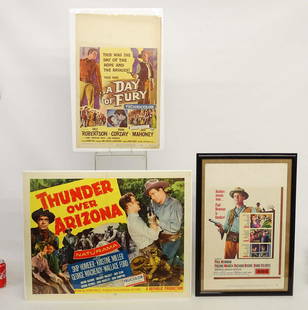The image showcases three vintage Western movie posters, all in distinct frames. The top left poster, titled "A Day of Fury," features a yellow and brown color scheme with a cowboy and an Indian cautiously peering around a corner. The print on this poster is difficult to read. Below it, the second poster, "Thunder Over Arizona," is highlighted with the title in bold red letters on a yellow background. It depicts a tense standoff with two armed figures aiming guns at each other, accompanied by an additional cowboy figure in the background. The third and final poster, positioned to the right and framed in black, portrays a sharply dressed cowboy wearing a hat and pointing a gun. The details on this poster's text are also too small to decipher. Notably, a recognizable red Coca-Cola can is partially visible either on a table or the floor beneath these displays. The posters seem to be showcased for a particular reason, possibly celebrating classic Western cinema.